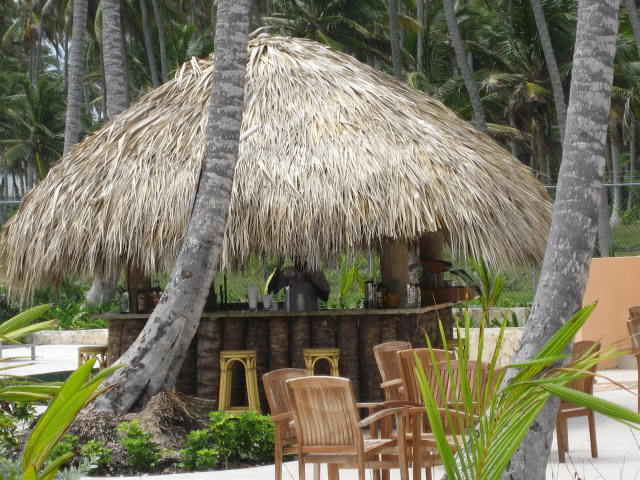This vibrant color photo captures a lively outdoor bar at a tropical resort, featuring a large Tiki hut made from bamboo and topped with a distinctive V-shaped grass roof. The hut serves as a bar and is surrounded by wooden tables and chairs arranged on a ground that appears to be sandy but smooth, suggesting it might be cement. Enclosed by lush palm trees, the scene feels secluded yet inviting, with a hint of water visible in the background to the left. The bar area is lively, with various cups and bottles displayed, and a bartender— a black man in a gray short-sleeve shirt—busily preparing drinks. The bartender appears to be shaking up a concoction, adding to the dynamic atmosphere. This well-crafted Tiki hut scene is a bustling social spot amidst a picturesque tropical island resort.